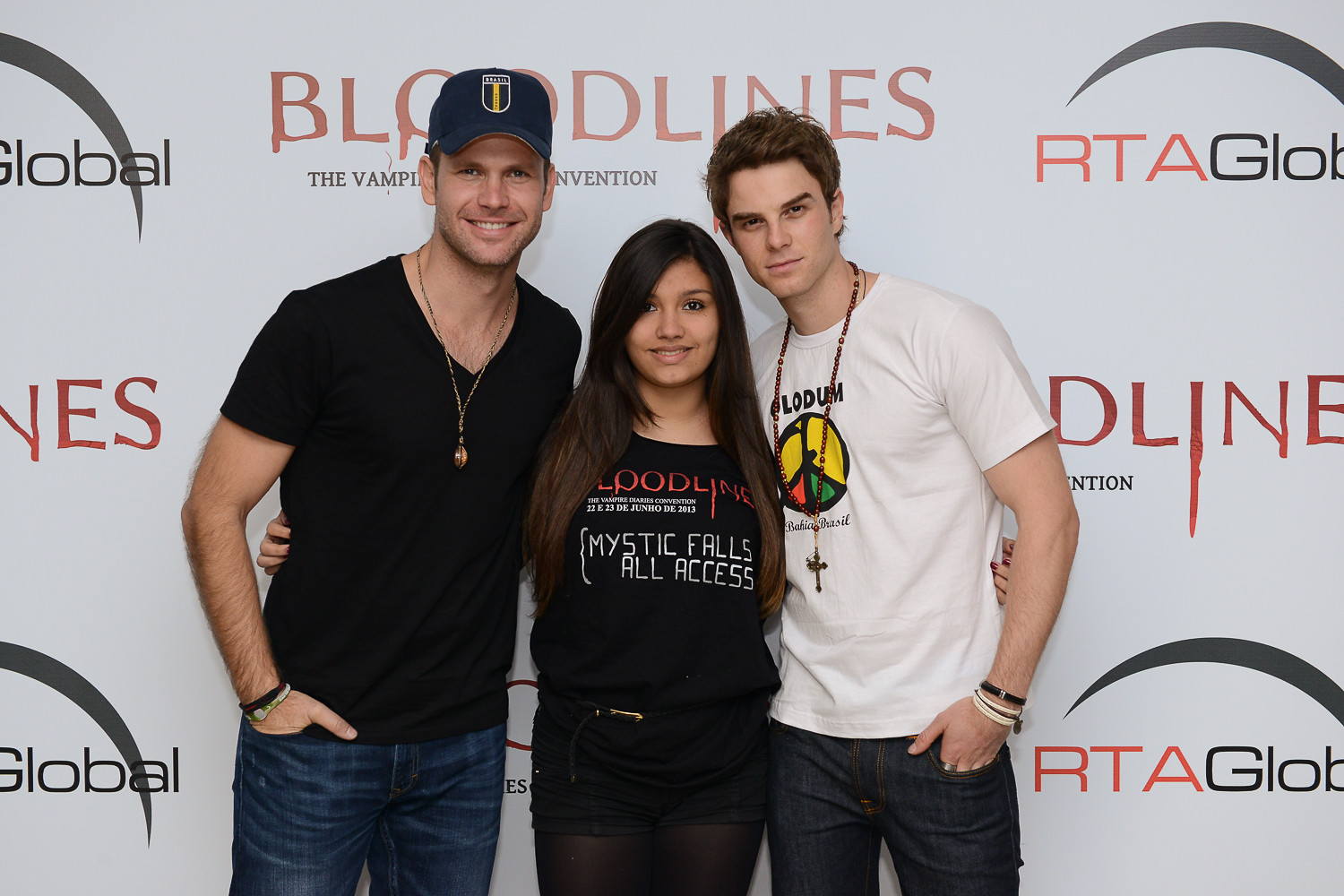In this photograph, taken indoors against a light grey wall adorned with repeating logos that read "Bloodlines," "The Vampire Convention," and "RTA Global," three individuals are centrally positioned, smiling directly at the camera. The backdrop's repeated red and black text signifies a promotional event for the Vampire Bloodlines Convention.

In the center of the image stands a young woman with light tan skin and long brown hair, partially trimmed at the shoulders to create long bangs, and flowing down to mid-chest. She is wearing a black t-shirt emblazoned with "Bloodlines" in red and "Mystic Falls All Access" in white, paired with dark black shorts over black tights.

To her left is a tall man of Caucasian descent, donning a blue ball cap, a short-sleeved black shirt, and a gold necklace with a small pendant. He has one hand in his jeans pocket and the other arm around the woman's shoulder. On her right is a younger man, also Caucasian, with messy brown hair. He sports a white short-sleeved t-shirt featuring a peace sign, a beaded rosary necklace, and dark blue jeans. The trio is clearly at ease, embodying the spirit of the convention they are attending.